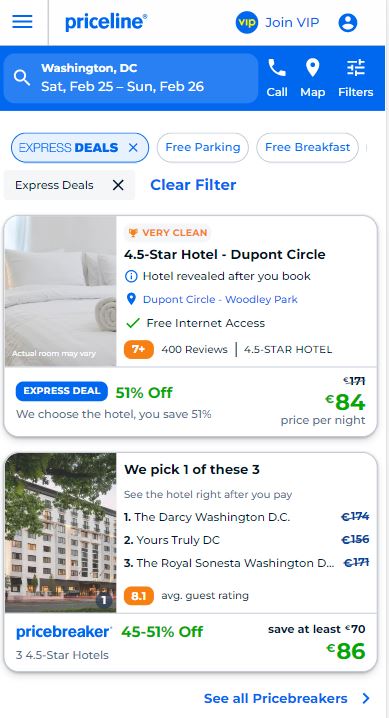The image, captured on a cell phone, displays a Priceline search for hotel accommodations in Washington, D.C. from Saturday, February 25th to Sunday, February 26th. The user has selected the "Express Deals" filter, which shows discounted rates while withholding the hotel's name until after booking. They also had the options to choose filters like "Free Parking" or "Free Breakfast," but those are not selected.

Two hotels appear as options under the "Express Deals." The first listing is a 4.5-star hotel in the DuPont Circle or Woodley Park area, labeled with "Hotel revealed after you book." This hotel offers free internet access and has received 7+ ratings from over 400 reviews. Currently, the express deal offers a 51% discount, reducing the price from £171 to £84 per night.

Below this listing, there is a choice list stating, "We pick one of these three hotels," which includes The Darcy, Washington, D.C., Yours Truly DC, or The Royal Sonesta Washington D.C., with a rate of £86 per night.